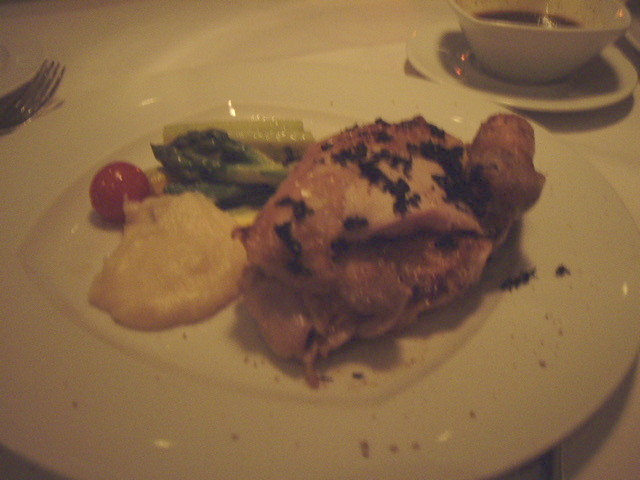The image depicts a dimly-lit photograph of a dining setting with a white tablecloth. Central to the frame is a large, circular white plate with a recessed center, filled with a main course that appears to be a piece of fried chicken, either a breast or thigh. The chicken has a few patches where the batter has been pulled off, revealing some slightly burnt, blackened areas. To the left of the chicken, there is a small scoop of mashed potatoes, slightly yellowed due to lighting. At the back of the plate, a few stalks of asparagus are visible, and on the far left is a shiny cherry tomato. Just inside the left edge of the frame, the tines of a fork are observable. Behind the main plate, there is another serving plate with a cup of coffee. The image is slightly out of focus, suggesting it was taken with a lower quality camera. The overall ambiance is dim, making the details harder to distinguish.